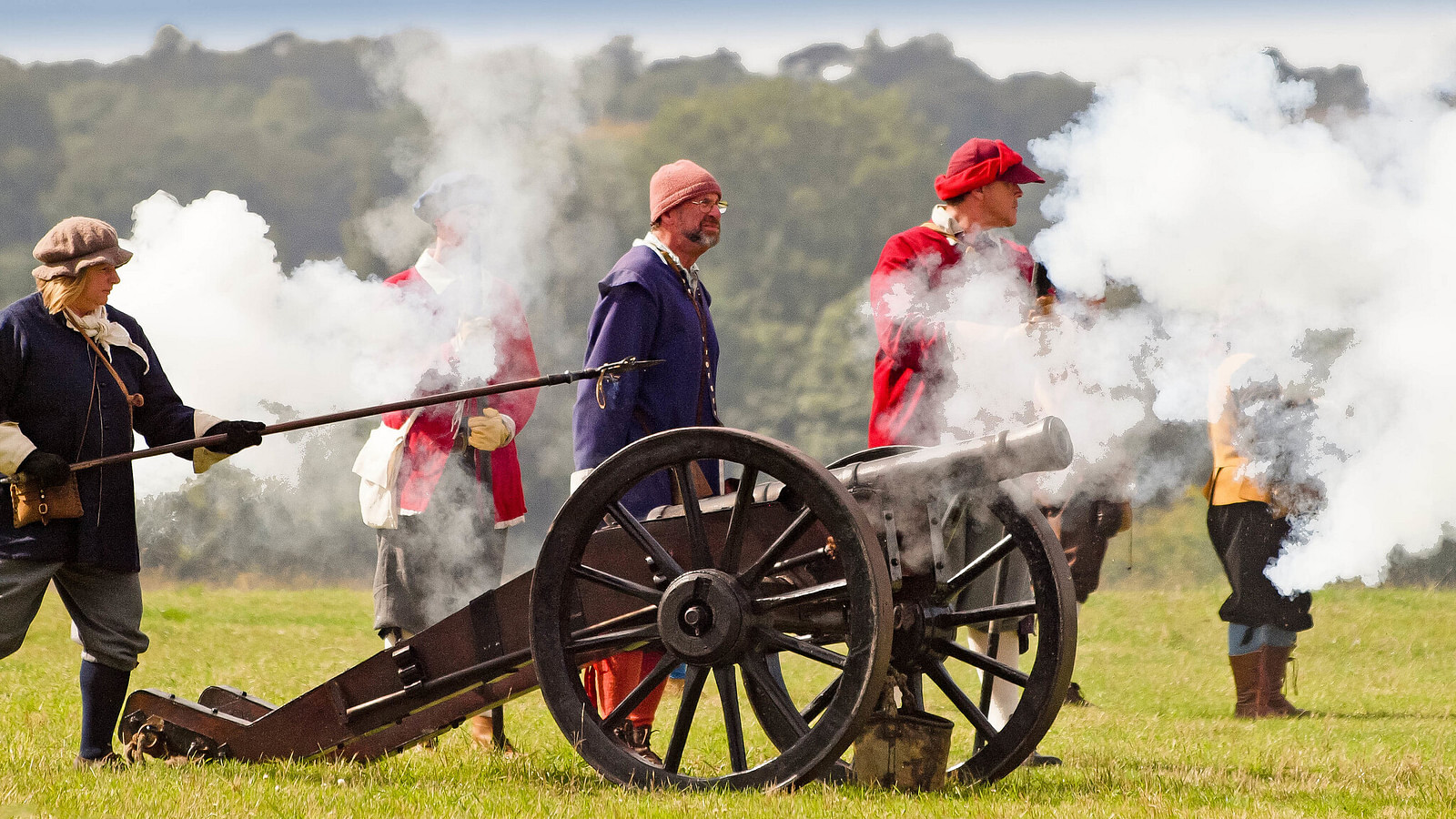The photograph, set horizontally, captures a detailed scene of a historical reenactment on a lush green grass field, bordered by trees in the background with a hint of sky peeking through. Central to the image is an antique cannon, reminiscent of those used two to three hundred years ago, mounted on wooden wheels. The area is enveloped in smoke, suggesting a recent cannon firing. The individuals in the scene, dressed in clothing typical of the colonial European era, include four men in a mix of red and blue jackets and a woman on the left holding a long stick, likely used to light the cannon. The attire includes poofy pants, frilly collars, and historical hats. The man at the center wearing glasses and a blue jacket gazes forward in the direction of the cannon, embodying the serious demeanor of the portrayed period. Their old-timey boots and detailed costumes, coupled with the smoky atmosphere, lend authenticity to the reenactment of an ancient British battle.